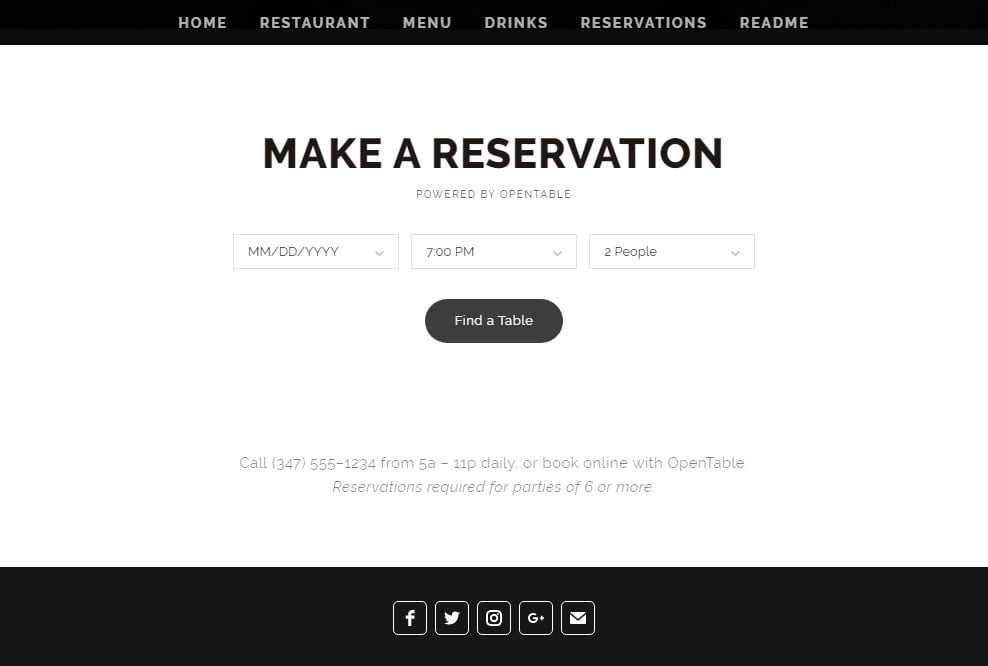The image displays a screenshot of a restaurant's online reservation page. At the top, a black header features a light gray menu with the options: Home, Restaurant, Menu, Drinks, Reservations, and Read Me. Below the header, bold large black text prominently reads "Make a Reservation" against a white background. Underneath, small light gray text states "Powered by OpenTable."

Three input fields are positioned beneath this text for making a reservation: the first field allows users to select the month, day, and year from a dropdown menu. To its right, another dropdown menu lets users choose their desired time, defaulting to 7 p.m. The third dropdown menu is for selecting the number of people, displayed as "Two People."

Below these fields, a prominent black action button labeled "Find a Table" invites users to proceed with their reservation. Underneath this button, light gray text provides additional information: "Call 347-555-1234 from 5 a.m. to 11 p.m. daily, or book online with OpenTable. Reservations required for parties of six or more."